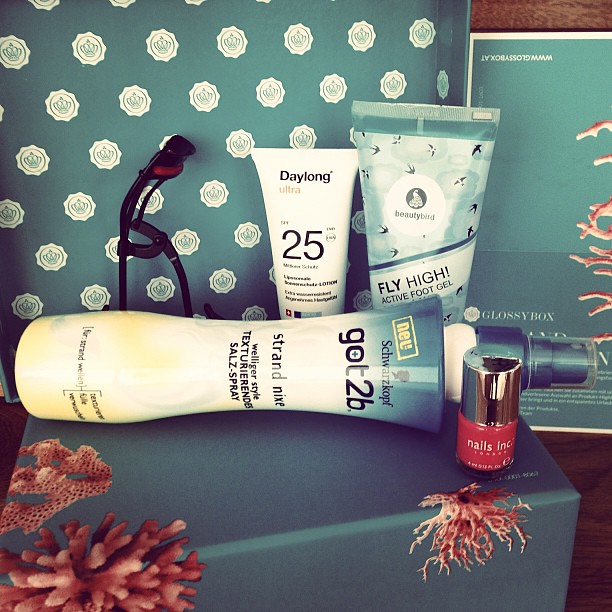The image depicts an open gift box with an assortment of beauty products arranged neatly inside. The box, labeled "Glossy Box," features a vibrant green background adorned with white spots. Inside the box, there's a collection of items including a "Day Long 25" product, a "Dot 2B" item, a "Fly High Active Foot Gel," and a bottle of nail polish. Scattered around the products are small pots of confetti and coral wreath decorations. Additionally, a twirly microphone can be seen in the background, adding a whimsical touch. The front corner of the box displays another coral wreath, complementing the festive and celebratory theme of the arrangement.